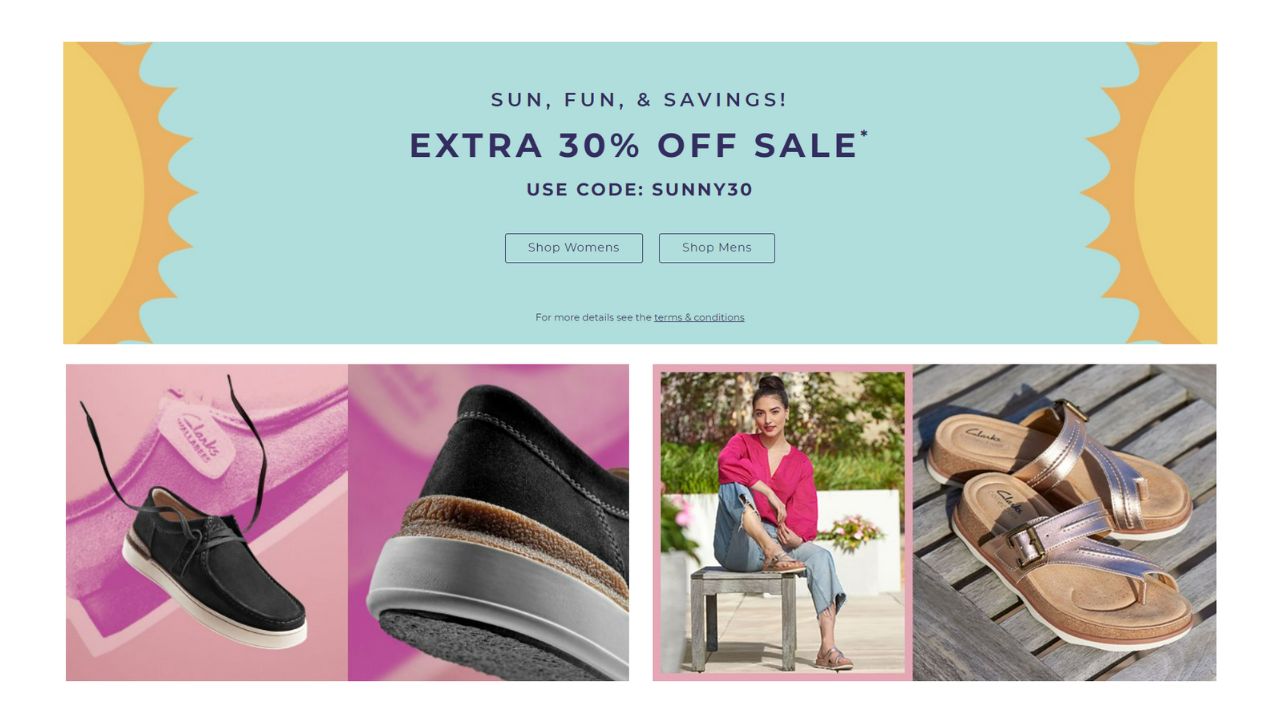This advertisement screenshot features a vibrant and summery theme. The top half of the horizontally rectangular image boasts a light blue background, reminiscent of a clear sky, with whimsical illustrations of the sun on both the left and right sides. These suns are depicted as yellow semicircles with bright orange rays radiating outward. Centered in this blue section is navy blue text that exclaims, "Sun, Fun, and Savings!" followed by "Extra 30% off Sale* Use code SUNNY30." Beneath this promotional message, there are two clickable rectangular buttons labeled "Shop Women's" and "Shop Men's." A note informs viewers to see the terms and conditions for more details.

The bottom half of the image is composed of a series of four distinct photographs. The first on the far left showcases a pale pink background with a hot pink shoe and a black shoe positioned in front of it. The adjacent photo highlights a similar hot pink shoe in the background, with a close-up focusing on the heel of the black shoe. White space separates this imagery from the next photograph. The third image features a woman dressed in calf-length denim pants and a hot pink three-quarter sleeve shirt. She has her long, dark hair styled in a bun and is seated outdoors on a bench, near a large planter filled with greenery. The background suggests the presence of a beach and additional plants. The final image on the right shows a rustic setting of what looks like a wooden deck or boardwalk, where a pair of sandals with brown soles and rose gold straps are placed.